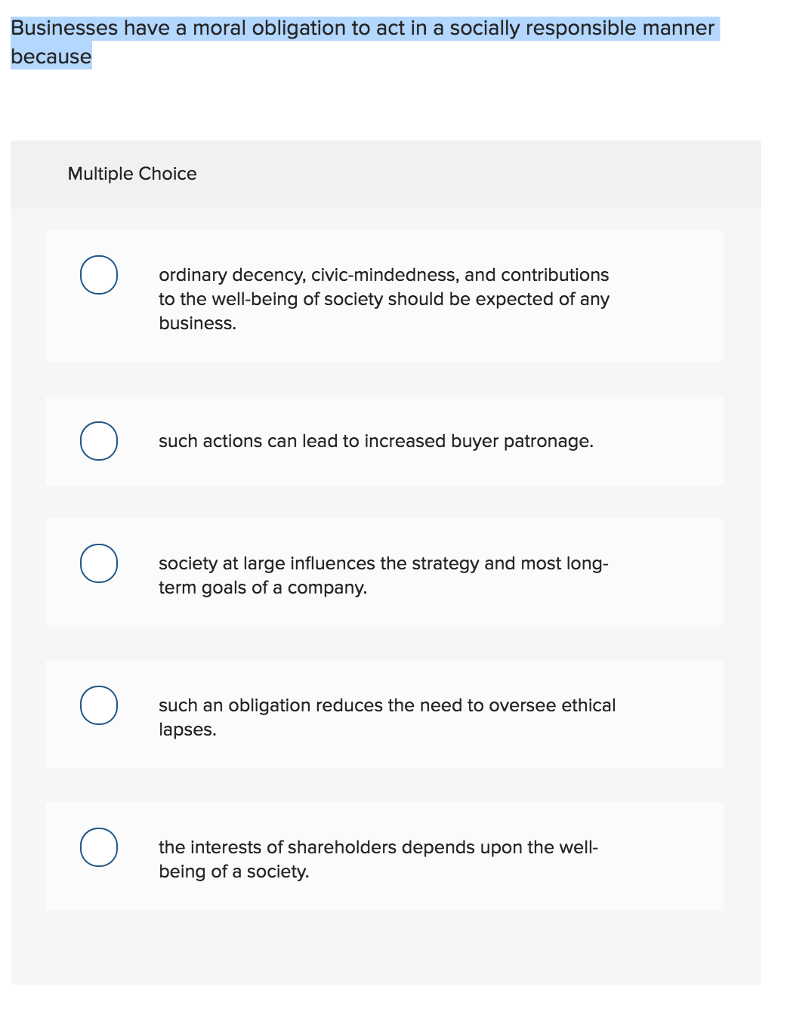The image is a minimalist white square background featuring a centered multiple-choice question without the question itself being shown. The text is uniformly small and black, with all elements neatly aligned. At the top left corner, the label "Multiple Choice" is displayed. Beneath it are five possible answers, each preceded by a blue-outlined circle:

1. "Ordinary decency, civic-mindedness, and contributions to the well-being of society should be expected of any business."
2. "Such actions can lead to increased buyer patronage."
3. "Society at large influences the strategy and most long-term goals of a company."
4. "Such an obligation reduces the need to oversee ethical lapses."
5. "The interests of shareholders depend upon the well-being of a society."

These responses are arranged vertically, each option positioned to the left of a circle. The simple and clean design emphasizes clarity and focus on the provided answers.